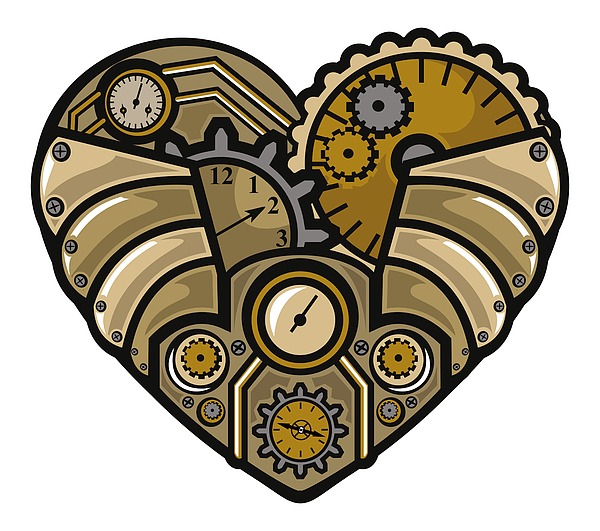This image is an intricate computerized drawing of a heart shape bordered by a thick black outline. The heart is filled with a complex arrangement of clocks, gears, and mechanical cogs, giving it a machine-like appearance. Predominantly colored in shades of brown, ranging from chocolate brown to light beige, as well as cream, blue, and black, the artwork intricately details various timepieces and mechanical elements. 

In the upper left-hand corner, there is a speedometer with a cream background and multiple borders in black, tan, and black again, set against a brown backdrop. The upper right-hand corner features a cream cog and a greenish-brown donut-shaped gear with black markings, interspersed with a blue cog. Centrally, towards the left, a clock with a blue outer rim and black numbers is visible, while below it, in the center, lies another clock, cream-colored with a single hand. Flanking these central elements on both sides are more brownish cogs with cream borders, giving the composition a symmetrical balance.

At the very bottom of the heart is another clock, this one featuring a blue outer rim and an orangey-brown face with black hands. The entire drawing is adorned with various screws and fasteners, enhancing the perception of depth and structure, as if the elements are physically held together. In the heart's core, there is a mechanical aspect that includes a partial clock face with the numbers 12, 1, 2, and 3, and an arrow pointing at 2, further emphasizing the time-centric theme. The heart is designed in an abstract manner and looks like it might be AI-generated or created using a computer program, making it a visually compelling fusion of organic shape and mechanical intricacy.